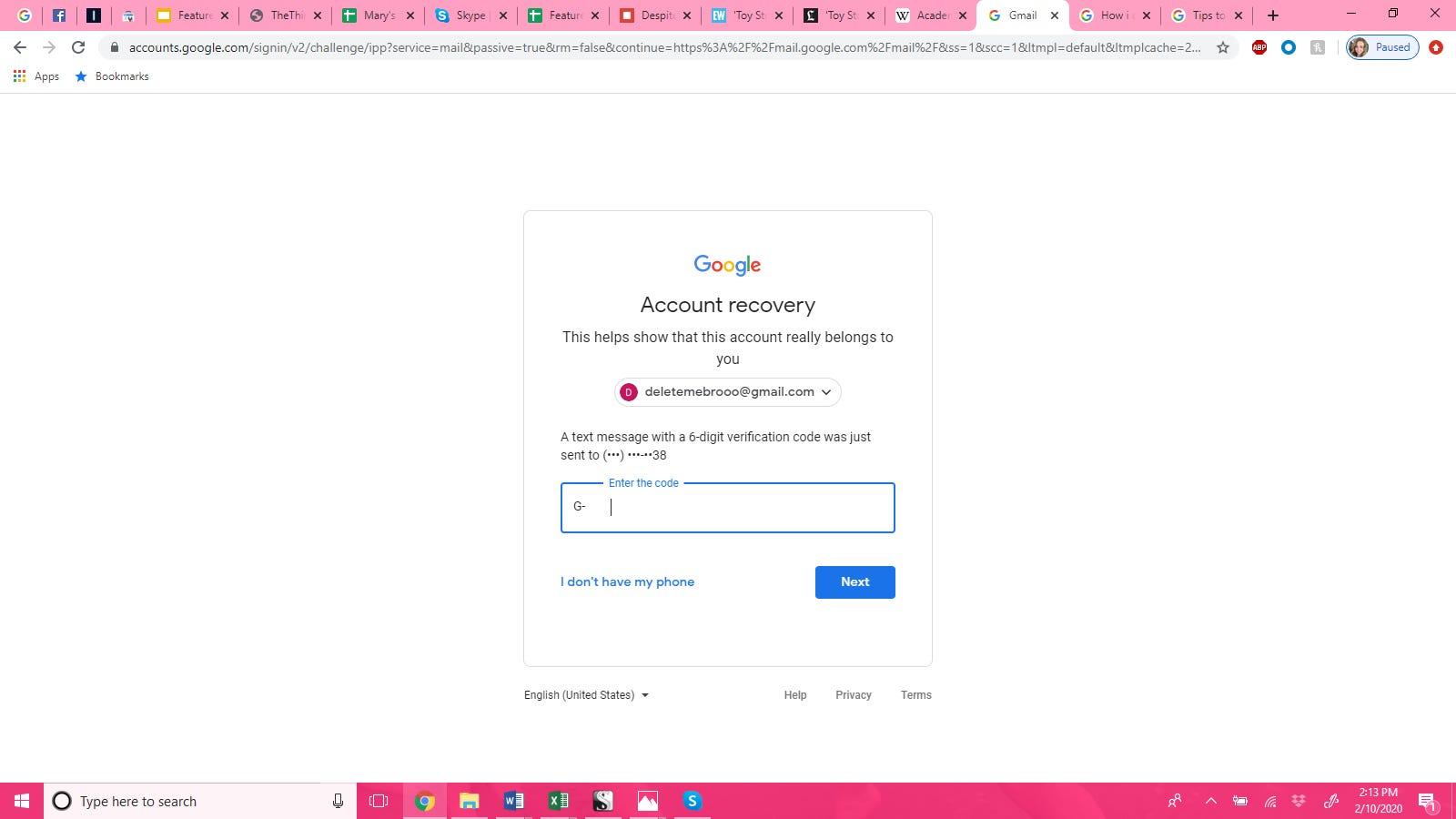*An Overlooked Digital Maze: A Google Account Recovery Journey*

The screen capture showcases a complex digital web in quintessential tech hues. Over the top, a substantial rectangular section is highlighted, reminiscent of a design by Google or Facebook. This area is bordered by an orange folder—possibly a sign of Mary's future digital landscapes intertwined with colorful icons.

At the heart of this maze is an intricate form resembling a never-ending code. The form oscillates between squares and arrows, leading to options like 'refresh', 'log in', and 'create account'. Embedded in this digital terrain is a URL strewn with a plethora of percent signs and slashes: HTTP://%3A%2Fcoma.gov.com/%2Fmail%2FFS=1.

The left sidebar displays an ominous red shield, denoting a paused bookmark, and a stark white screen urging the user to log in for Google account recovery. This interface proposes a gentle reminder that the account genuinely belongs to the user. A spread circle and a prompt for a six-digit verification code pops up, subtly whispering, "This is Google's verification."

Icons like a blue folder, green folder, and a Skype symbol pepper the backdrop. The gray toolbar at the bottom corner reads ‘2:30 PM’ and lists ‘October 10, 2020’. Simultaneously, a text box begs the user to "type here to search”, epitomizing a routine yet vital aspect of troubleshooting in our tech-driven age.